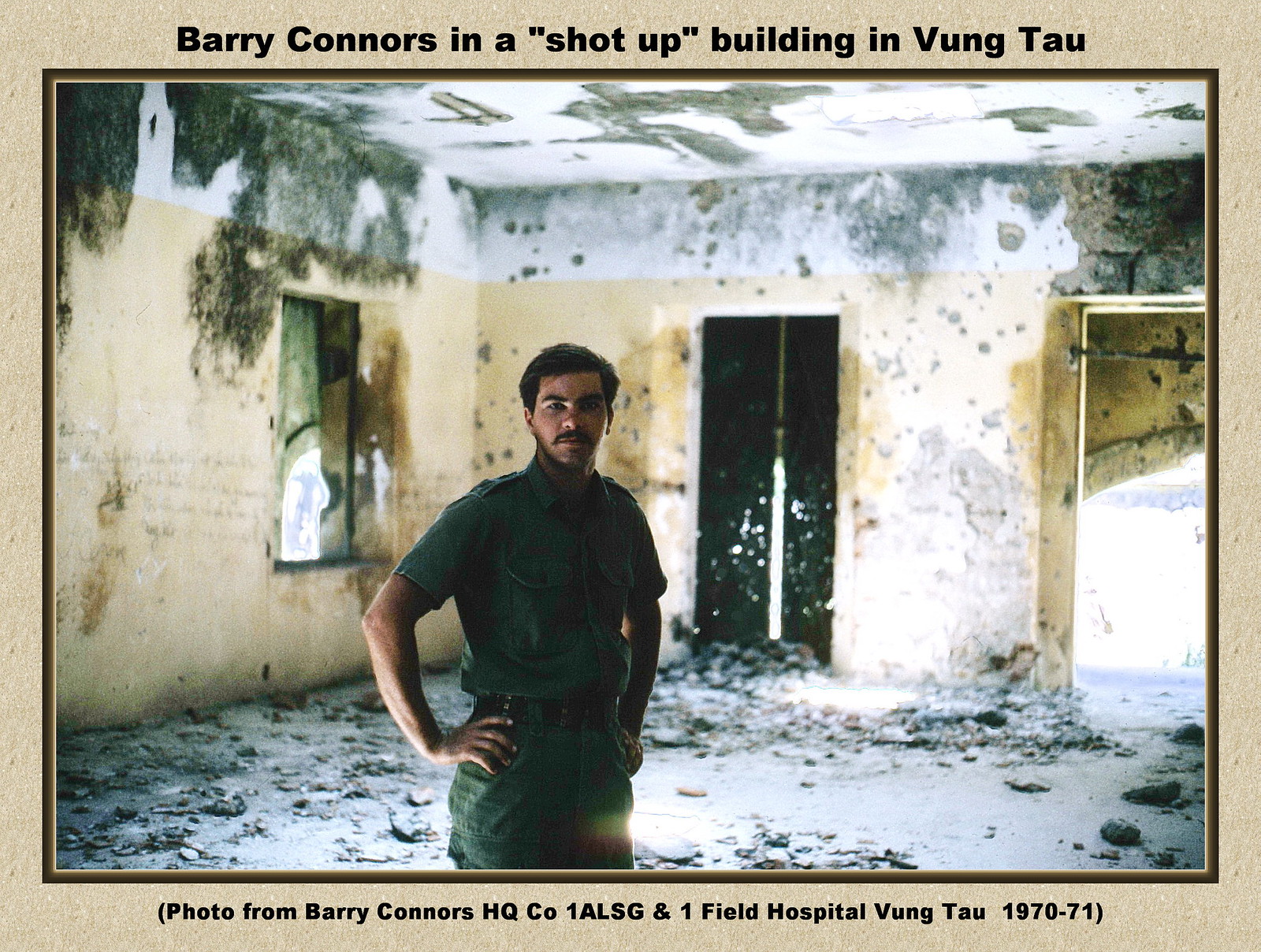The photograph captures a young man, identified as Barry Connors, standing inside a severely damaged building in Vung Tau, taken during the years 1970-71. Barry, likely in his 20s, is dressed in green military attire consisting of green pants and a short-sleeved shirt. He has dark hair, a mustache, bushy eyebrows, and dark eyes, which are directed towards the camera. The building, possibly a field hospital, shows signs of extensive destruction with decaying floors and ceilings, large black patches, broken windows, and concrete debris scattered on the floor. Bullet holes and dirt marks punctuate the battered walls, creating a stark, somber atmosphere. The inscription above the photo reads "Barry Connors in a 'shot-up' building in Vung Tau," and beneath the photo, it states, "Photo from Barry Connors, HQ Company 1 ALSG and 1 Field Hospital, Vung Tau, 1970-71." The photo itself is accented with a brown frame and a tan border.